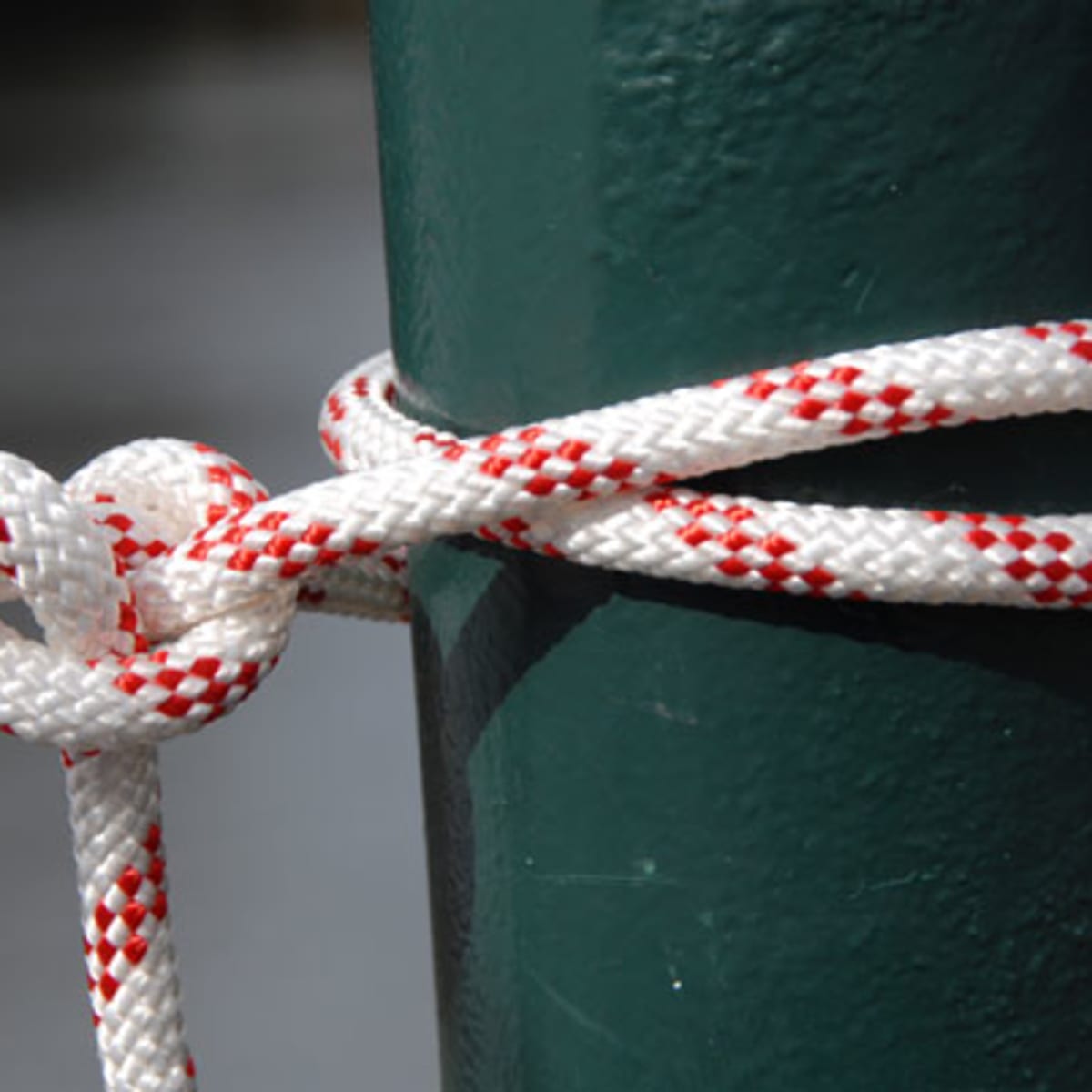The image is an outdoor photo depicting a thick, white rope with red stripes tied in a pretzel knot around a large, dark green pole. The pole, which takes up about three-quarters of the right side of the image, is partially cropped out, obscuring its full size. The background on the left side is a blur of light gray and black. The red and white colors on the rope alternate in each section, and the end of the rope hangs downward on the left side of the image. The overall composition emphasizes the contrast between the new, brightly colored rope and the dark, weathered pole.